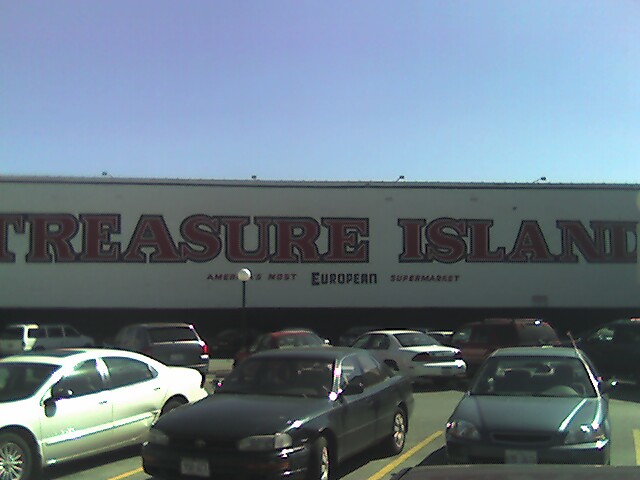The photo, taken likely in the late 1990s or early 2000s, shows the exterior of a supermarket called Treasure Island, located in a parking lot under a clear, sunny sky with no clouds. The image captures several cars, mostly sedans, parked diagonally. In the foreground, there are three cars facing the camera: a white sedan on the left, followed by two black sedans. Behind this row, another set of cars is parked diagonally in the opposite direction, including an SUV and mini SUVs. A lamppost with a circular light is also visible. The supermarket's sign is prominently displayed: "TREASURE ISLAND" in large red capital letters, partially cut off on the left side, followed below by the tagline "AMERICA'S MOST EUROPEAN SUPERMARKET," with "AMERICA'S MOST" in red, "EUROPEAN" in black, and "SUPERMARKET" again in red. The bright blue sky occupies the upper third of the image, highlighting the clear midday atmosphere.